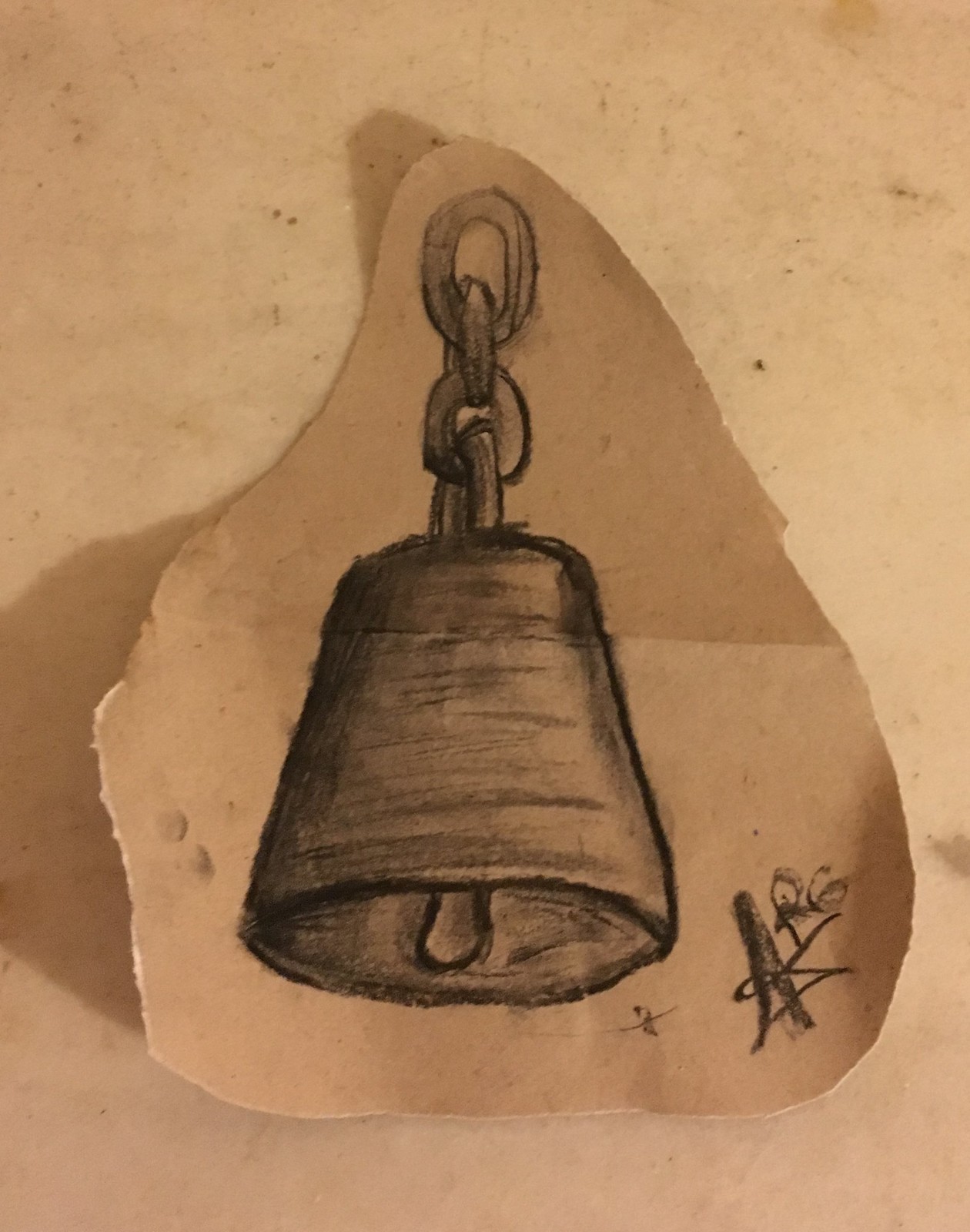The image features a hand-drawn bell on a peach-colored piece of paper. The background surface, resembling a pink table, is smudged with dirt. The bell was meticulously drawn in pencil and then cut out, leaving a thin border around it. The bell itself has a simple design, consisting of a circular base with sides that slope upwards slightly, outlined in black. Horizontal lines of shading, more concentrated on the left side, add a sense of roundness to the bell. A small clapper hangs down to represent the ringer. The bell is depicted as if suspended by four chain links at the top. In the bottom right corner of the image, the artist has signed their work with what appears to be the initials "A.G."